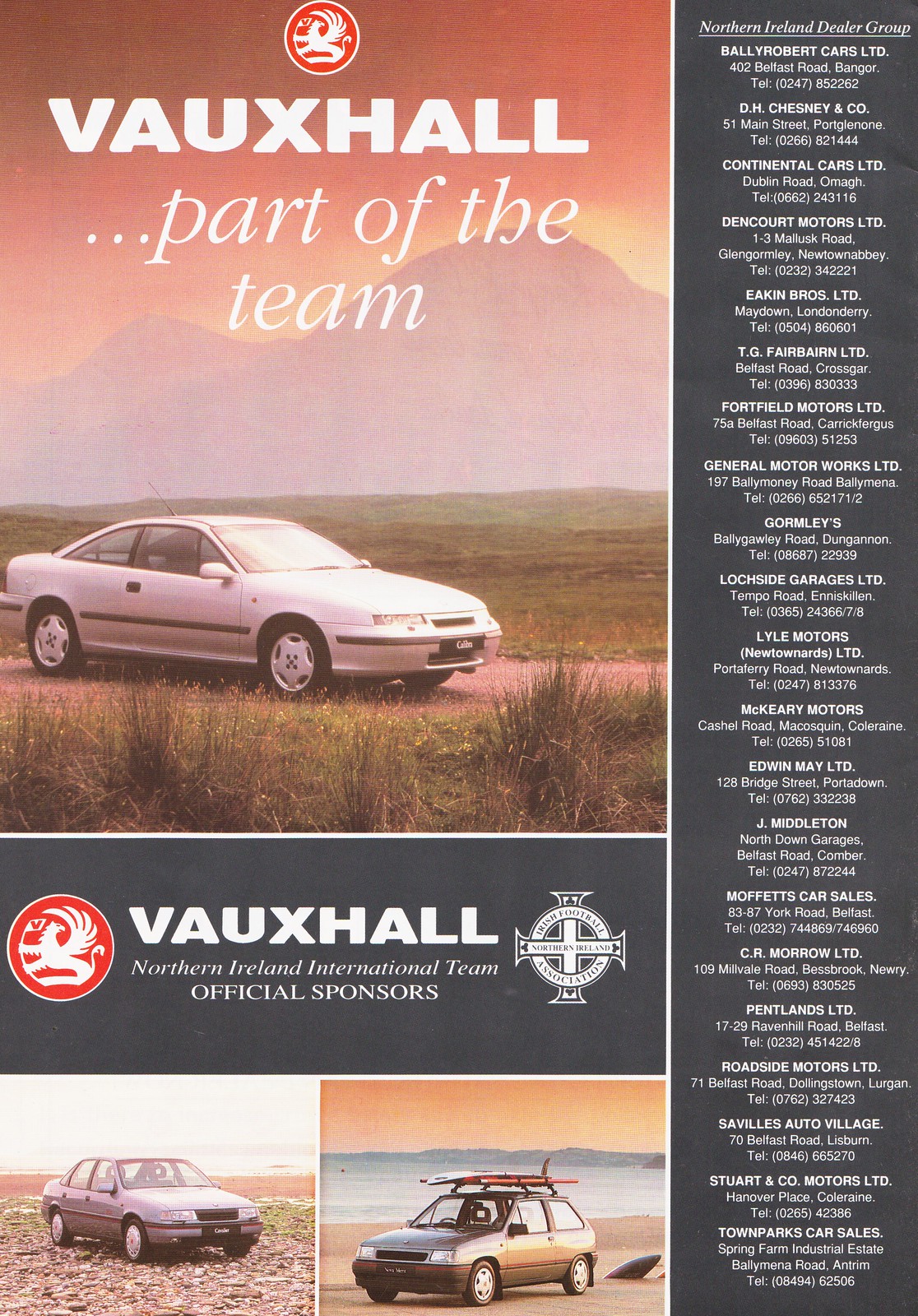This is a highly detailed Vauxhall car advertisement, likely intended for a magazine given its vertical, rectangular dimensions. The central focus is a striking image of a silver, two-door Vauxhall car positioned on a road amidst a mountainous landscape. The top of the image features the Vauxhall logo, a red circle with a white griffin holding a flag, followed by bold white text reading "Vauxhall" and the slogan "part of the team."

The advertisement also highlights Vauxhall's official sponsorship of the Northern Ireland International Team, with this designation prominently displayed on a dark grey background beneath the main car image. Here, the text includes "Vauxhall Northern Ireland International Team Official Sponsors" alongside the Irish Football Association's logo.

The right-hand section of the ad lists various Northern Ireland dealership locations, emphasizing the manufacturer's extensive network. Additionally, the lower segment showcases two smaller car images: one of a four-door sedan on the left and another of a two-door hatchback on the right, further illustrating Vauxhall's range of models. The overall composition is meticulously designed to highlight both the brand's premium vehicles and its community involvement.